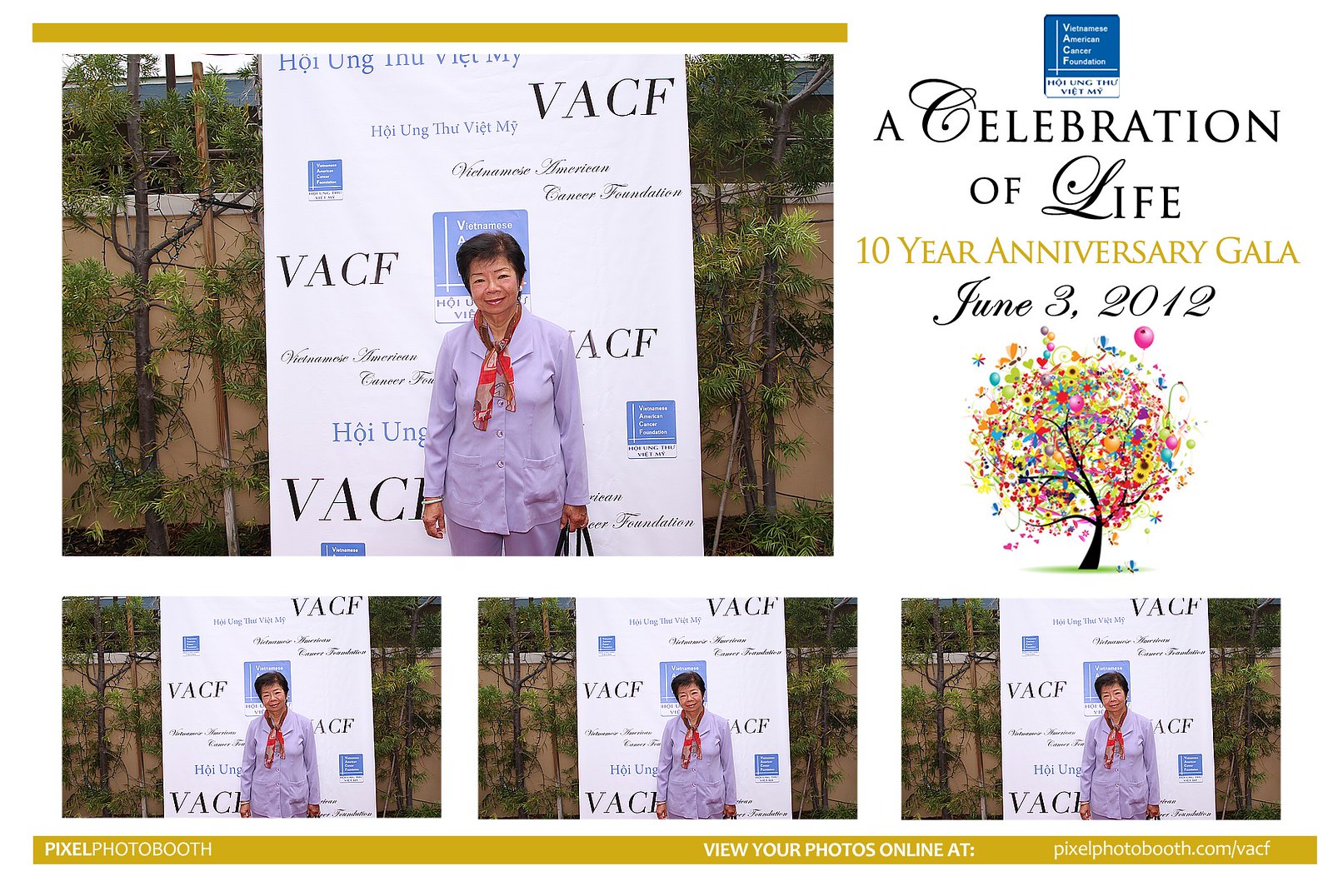This image features an older Asian woman with short cropped black hair, dressed in a coordinated purple ensemble that includes a long-sleeved jacket and dress pants, complemented by a red and white scarf around her neck. She is holding a black purse and standing proudly in front of a press banner adorned with multiple logos, prominently featuring the Vietnamese American Cancer Foundation (VACF). The banner, which includes text written in Japanese and a blue and white logo, indicates her involvement in a cancer charity event. The background shows a wall with trees planted nearby. 

To the right of the woman, there's a white area of text which states, "Vietnamese American Cancer Foundation" and reads "A Celebration of Life, 10 Year Anniversary Gala, June 3, 2012" in various fonts and colors. Below this text is an illustration of a tree with leaves depicted in vibrant colors ranging from pink to blue to purple, interspersed with balloon illustrations, giving a festive feel to the image. At the bottom of the image, repeated photographs can be seen with the caption, "Pixel Photo Booth, view your photos online," suggesting that attendees could order their event photographs. This photo captures a moment of celebration at a significant charity event, commemorating a decade of the foundation's work.